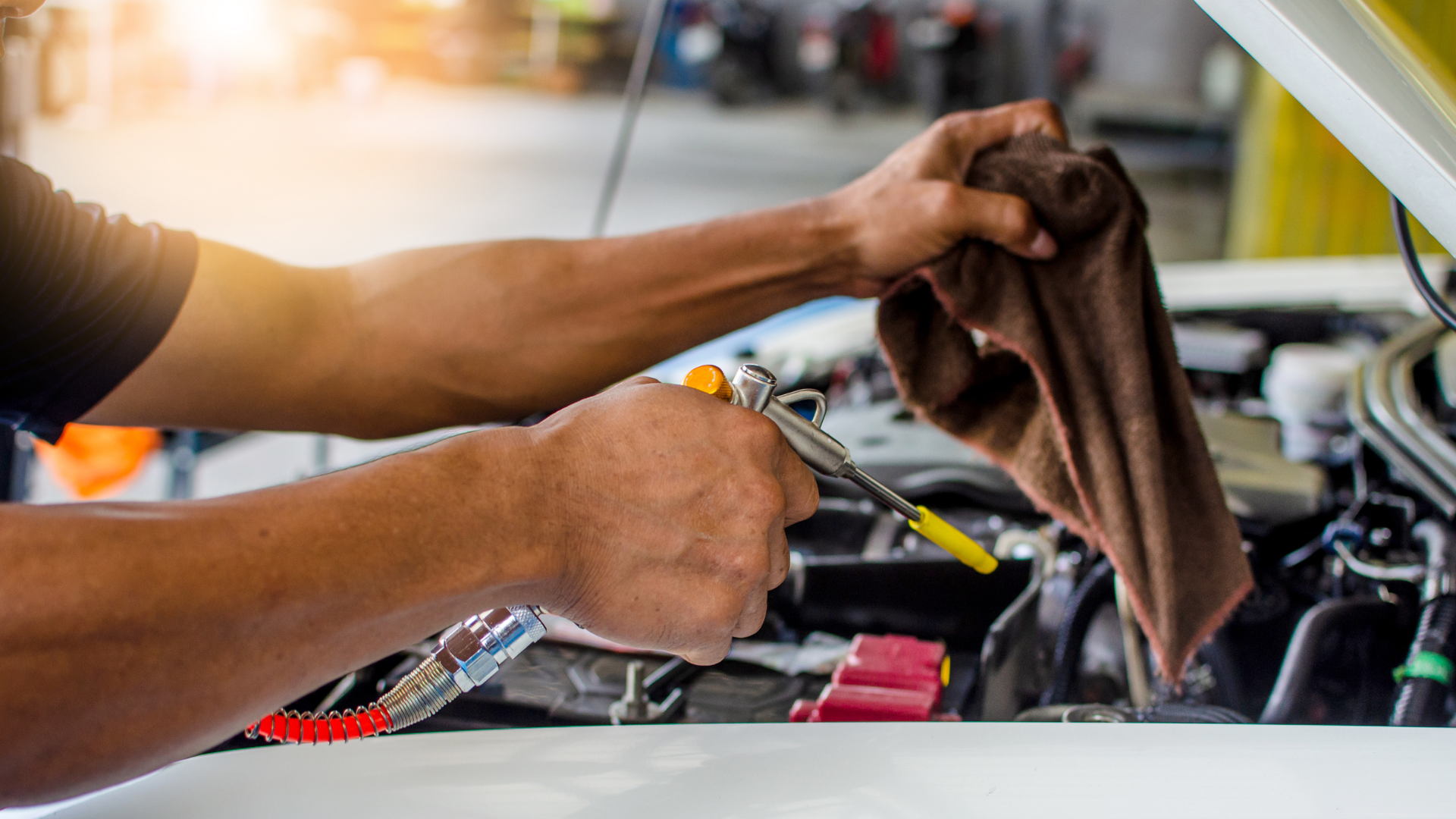In this color photograph, a mechanic is working under the propped-up hood of a car. The image is tightly cropped, revealing only the mechanic's arms from the biceps to the edge of the car on the right side. In his right hand, the mechanic holds a tool with a yellow edge, an extended rod featuring a red cord and silver fixtures, suggesting he is checking or refilling a fluid, possibly oil. His left hand clutches a brown rag, indicating the necessity for wiping or cleaning during the task. The brightly lit shop in the background is blurred and out of focus, emphasizing the action beneath the car's hood. No other people are visible, and the vehicle's make and model remain unidentified due to the limited view of the scene. The photograph's orientation is longer than it is tall, offering a detailed yet constrained glimpse into the mechanic’s diligent work on the vehicle.